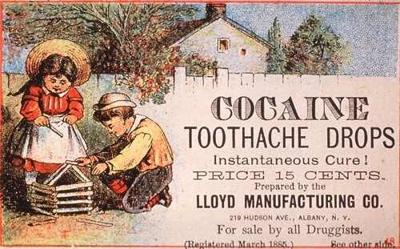This vintage illustration, likely a watercolor painting, showcases an early advertisement for "Cocaine Toothache Drops," promising an instantaneous cure for the price of 15 cents. Prepared by the Lloyd Manufacturing Company and distributed by all druggists, it dates back to March 1885. The scene features a little boy and girl engaged in building a small wooden house on the sidewalk. The girl, wearing a red dress with a white apron and a straw hat, has dark hair styled in a braid. The boy sports a yellow blouse, green pants, and a white hat. The background includes a white picket fence, a large green tree adorned with orange and red flowers, and a house with a blue roof. The detailed advertisement text is in large black letters, segmented to the right of the children, adding to the nostalgic charm and intriguing historical context of the image.